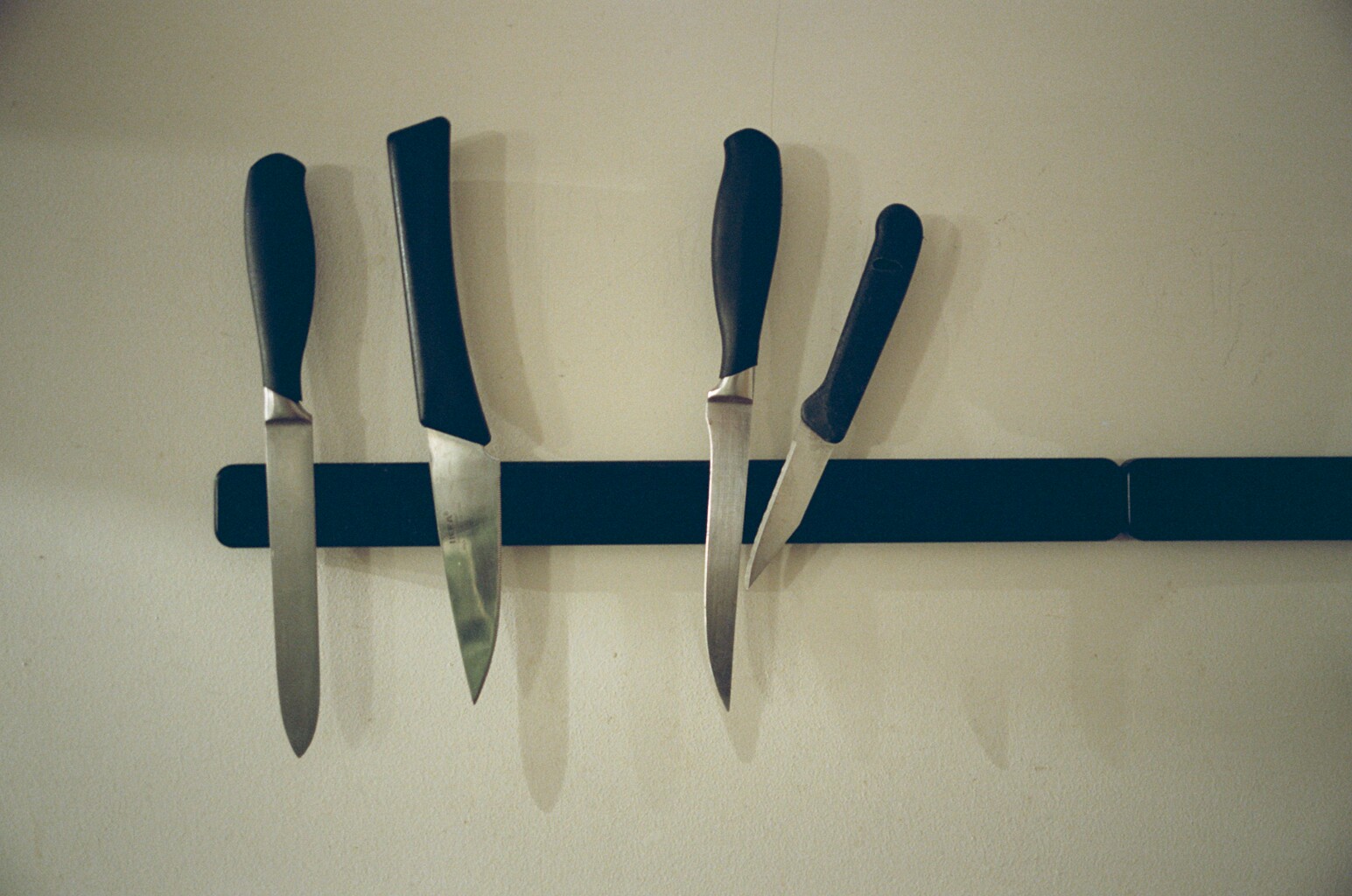This landscape-oriented photograph showcases a realistic scene featuring a nearly off-white wall with a slight hint of shadow, possibly from the lighting in the room. The focal point of the image is a series of black magnetic strips mounted horizontally across the center of the wall. Two strips are aligned in a continuation; however, only one is entirely visible, while the second one extends off the photo’s right edge, with a portion still in view.

Affixed to the fully visible magnetic strip are four stainless steel kitchen knives, all of which have black handles of varying ergonomic designs. The knives are displayed with their blades magnetically attached to the strip and their points facing downward. Each knife is distinct: the leftmost is tall and thin; the second is broader with a shorter blade; the third is smaller with a curvier design; and the rightmost resembles a paring knife, ideal for detailed cutting tasks. The scene is well-lit, accentuating the clean lines and blades' sharpness, as well as casting soft shadows on the wall, further enhancing the realistic details in the photograph.